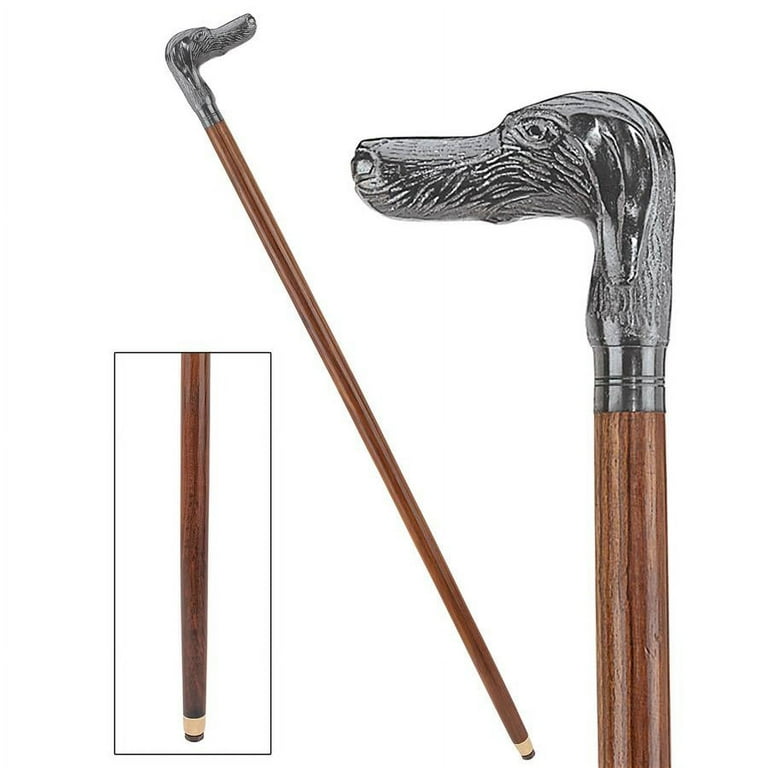The image displays three separate views of an ornate and unique wooden cane, placed side-by-side. On the left, a small inset image, bordered in black, highlights the lower portion of the richly dark wood cane featuring a white tip, reminiscent of a pool cue. The middle segment showcases the full length of the slender wooden cane, revealing its intricate craftsmanship. Attention is drawn to the handle—a detailed silver metal carving of a dog's head. The rightmost image offers a close-up of this silver handle, capturing the fine details of the dog's head, including its floppy ears, expressive eyes, and elongated snout. The combination of these images provides a comprehensive view of the cane's artistic elegance and functionality.